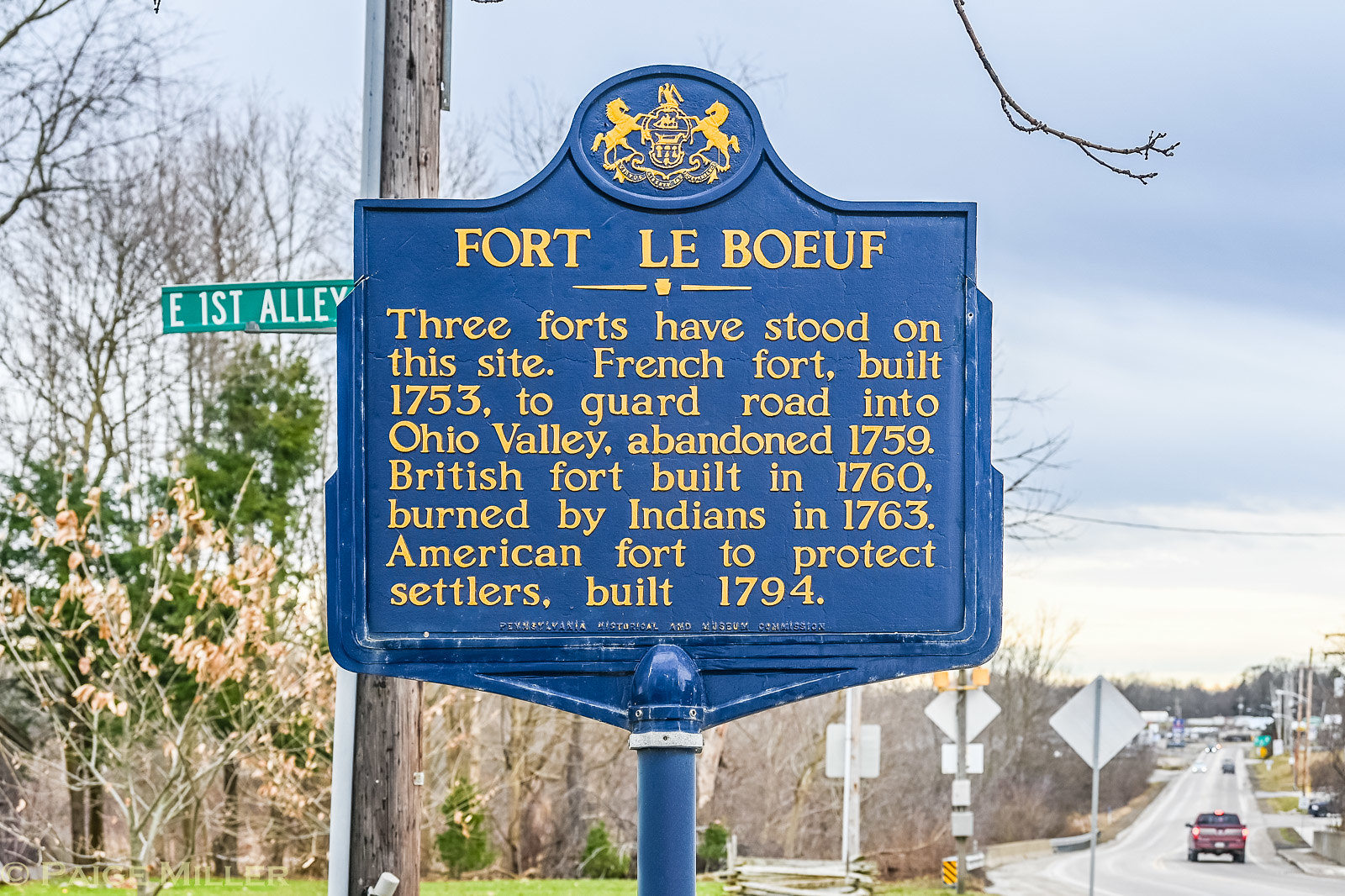The image depicts a prominent blue road marker, prominently featuring the words "Fort LaBeouf" in yellow letters. Erected on a blue pole, this plaque outlines the historical significance of the site, noting that three forts once stood there: a French Fort built in 1753 to guard the road into the Ohio Valley, abandoned in 1759; a British Fort built in 1760, burned by Indians in 1763; and an American Fort built in 1794 to protect settlers. At the top of the plaque, a detailed coat of arms is visible, showing two horses rearing against a shield topped by an eagle, though the accompanying banner's text is illegible. The marker is set against an outdoor backdrop that includes a street labeled "East First Alley" on a sign behind the marker. A road runs along the right side of the image, on which a red pickup truck can be seen driving away from the camera, with additional vehicles farther in the distance near what appears to be a small town. The scene is characterized by a mix of leafless and partially leafed trees, a blue sky with hazy clouds, and some patches of grass.